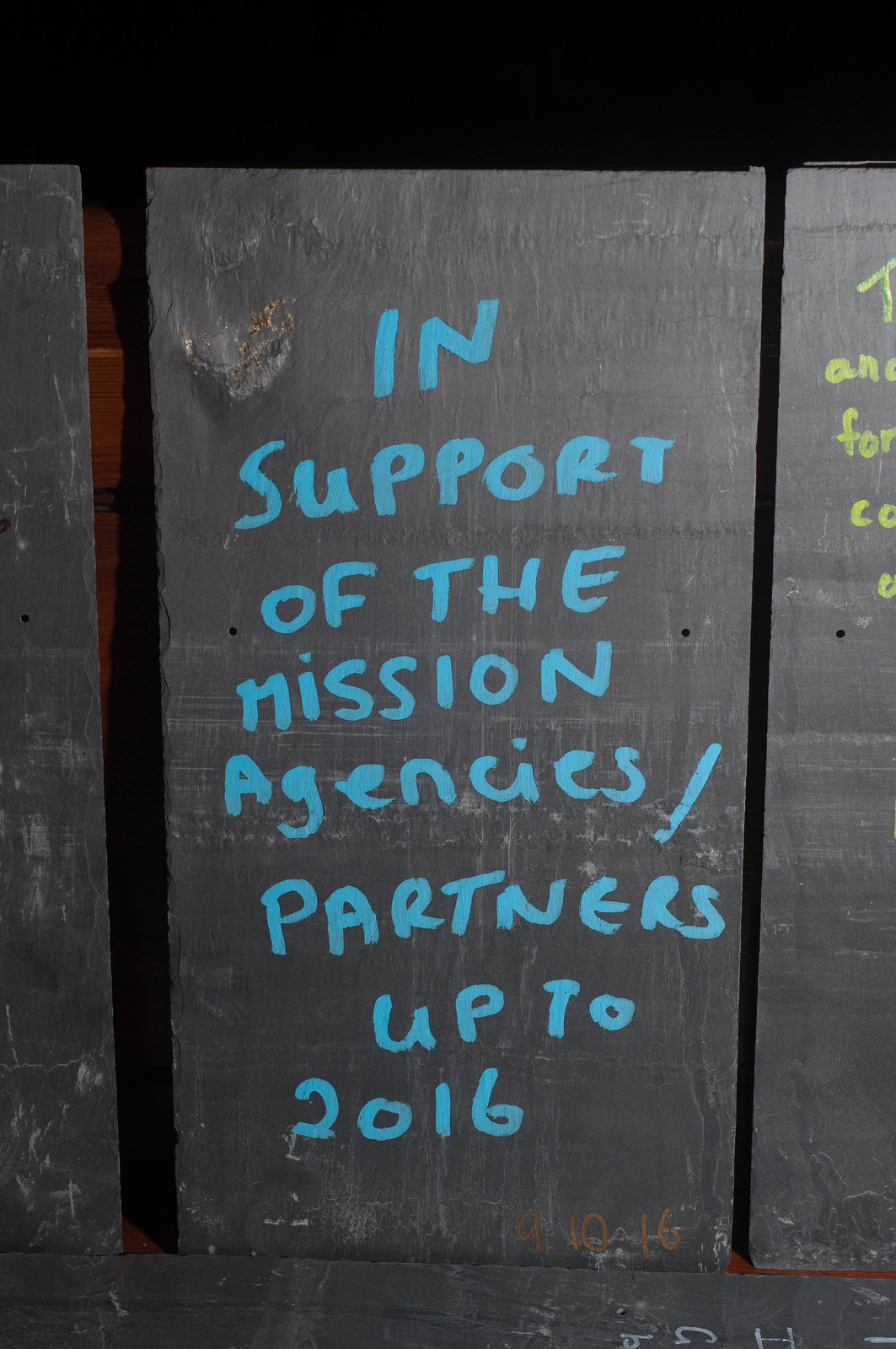The image presents a dark, slate-gray background resembling a weathered and jagged stone tablet, possibly made of actual slate. Positioned centrally, one distinct tablet features prominently, with others lined up beside it. This central tablet bears handwritten text in a light blue or turquoise hue, stating, "In support of the mission agency/partners up to 2016." Towards the bottom, partially obscured but visible, is a date written in a goldish-yellow text, reading "9, 10, 16." The setting appears to be outdoors, potentially at night, with a bamboo stick or wooden fence post visible on the left side, contributing to the rustic and aged ambiance of the scene.